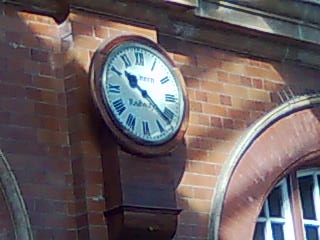The image depicts a close-up section of a brick building showing a clock mounted against a pillar. The building and the pillar are constructed from a combination of dark red and white bricks. The clock, which is round with a white face and black Roman numerals, is set within a dark brown, rectangular wooden base that attaches it to the brick pillar. The clock's hour hand, shaped like a wide arrow, is positioned between the 10 and the 11, and the longer, skinnier minute hand is between the 4 and the 5, indicating the time is approximately 10:21. The clock also features two unreadable words on its face, likely the brand. Above the clock, there is a small brown overhang. To the right of the clock is an archway bordered in brown, with a window beneath it. The window frames and panes are white and appear to be made of wood. The building is topped with a concrete border of a grayish-brown hue.